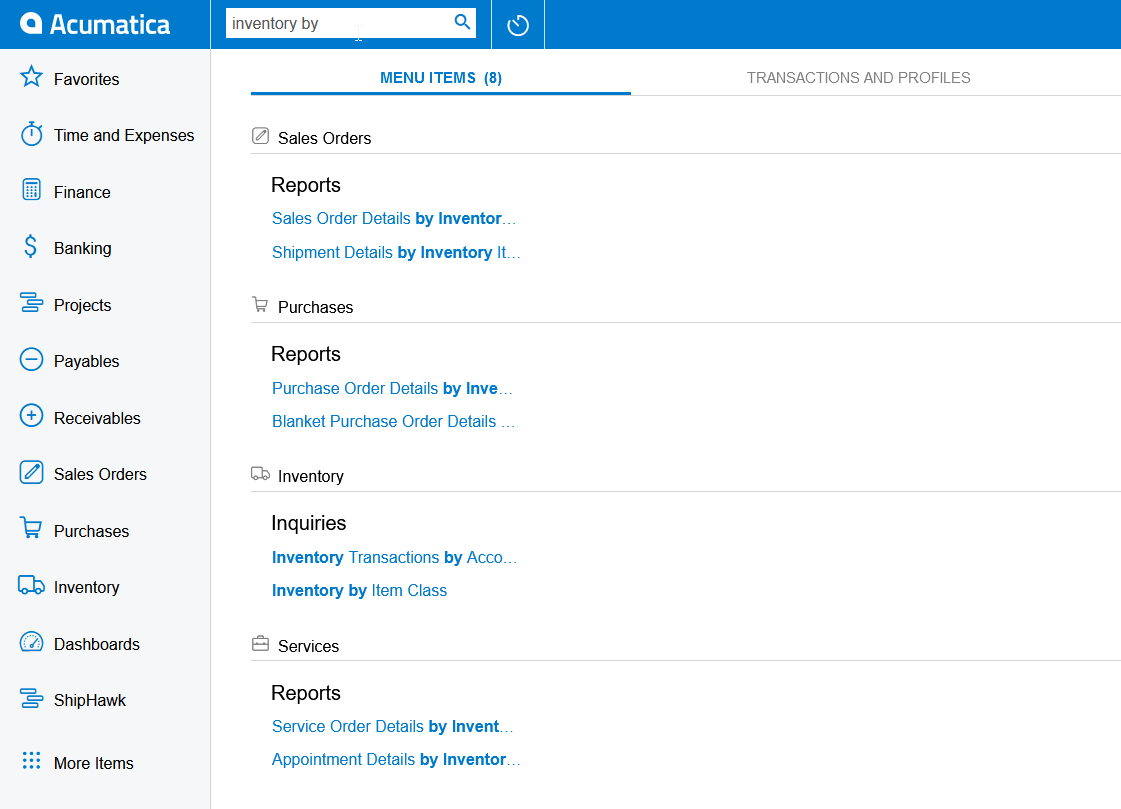The image displays a web page primarily in shades of white, blue, and black. At the top, a blue banner prominently features the word "AcuMedica" in white text. Below this banner, there is a search bar where the phrase "inventory by" has been entered. Adjacent to the search bar is a clock icon.

On the left side of the page, there is a vertical menu with various options, each accompanied by an icon:
1. **Favorites** - represented by a star.
2. **Time and Expenses** - illustrated with a stopwatch.
3. **Finance** - shown with a calculator.
4. **Banking** - identified with a dollar sign.
5. **Projects** - marked by three horizontal lines.
6. **Payables** - depicted with a circle containing a minus sign.
7. **Receivables** - illustrated with a circle containing a plus sign.
8. **Sales Orders** - shown with a square box and pencil icon.
9. **Purchases** - represented by a shopping cart.
10. **Inventory** - depicted with a truck icon.
11. **Dashboards** - marked by a clock icon.
12. **ShipHawk** - identified with three stacked rectangles.
13. **More Items** - illustrated with nine small dots.

The "Menu Items" section is highlighted in blue. Within this section, "Sales Orders" and "Reports" are displayed in black text. The sub-menu item "Sales Order Details by Inventory" is shown in blue, indicating it has been selected.